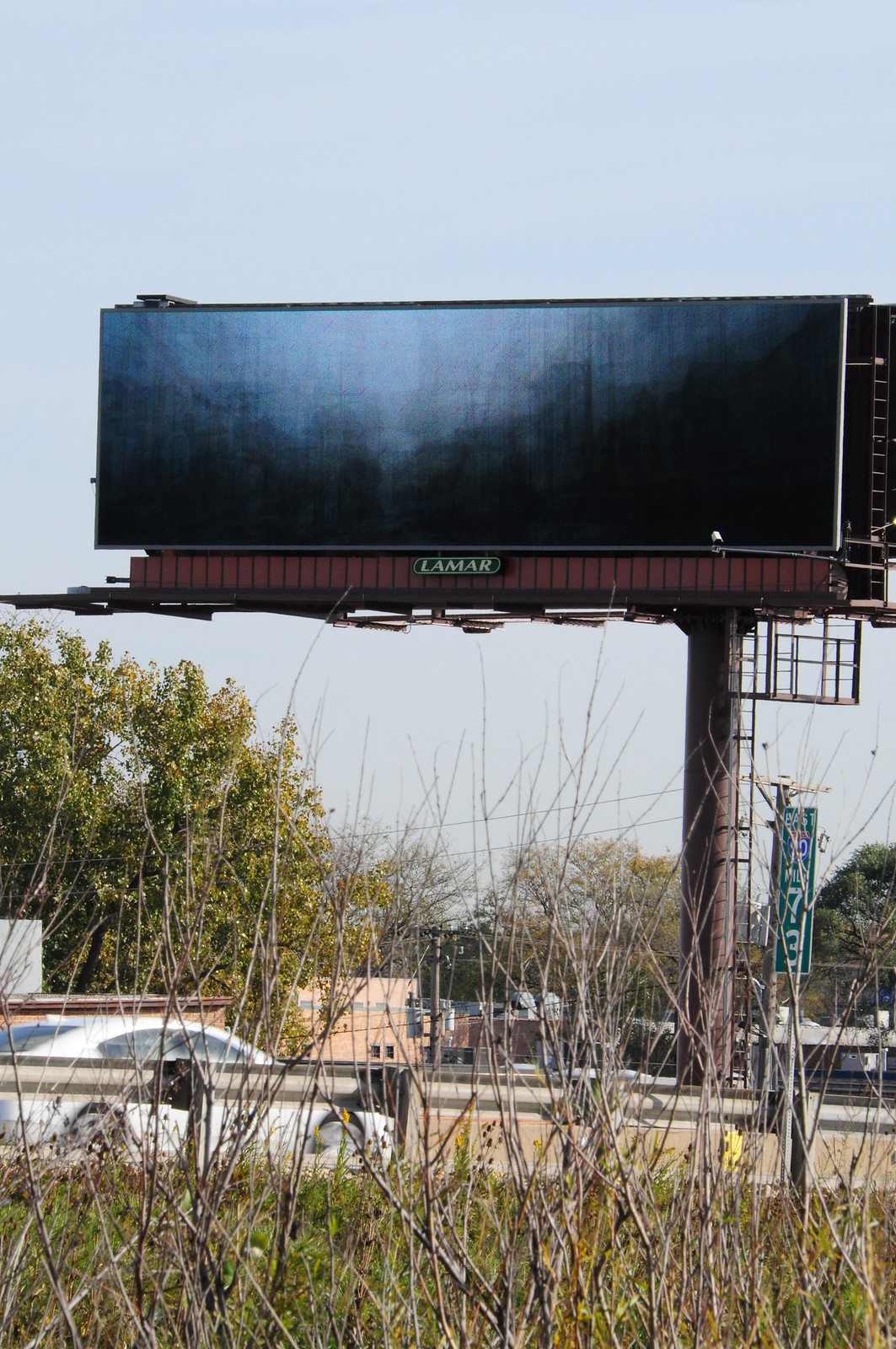A daytime photograph captures a unique billboard, mounted on a structure resembling a black freight container commonly seen on cargo ships. The container appears to have an open door on one end, although this is not entirely clear. The front of the billboard is painted burgundy and prominently displays an oval green plaque with the word "Lamar" written in white letters. The scene is set on a sunny day, with various types of brush and vegetation surrounding the area. In the background, a mile marker sign is visible, indicating either 73 or 78, suggesting proximity to an interstate. Trees and weeds are also present, further emphasizing the location's roadside environment.